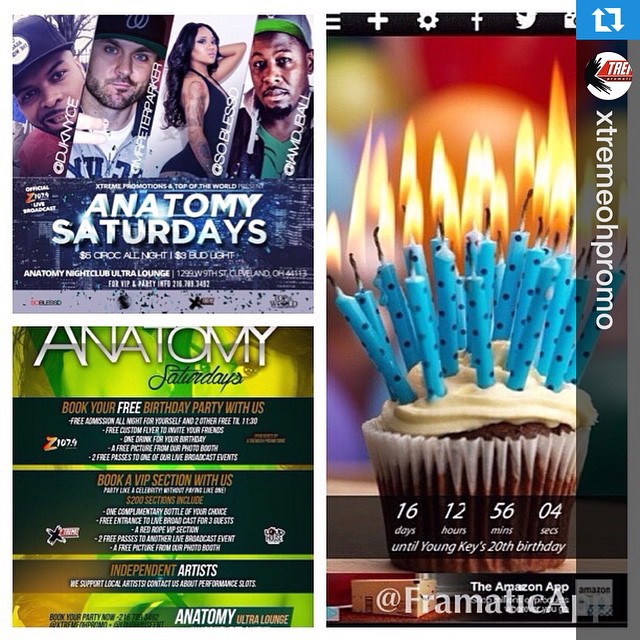The image is a vibrant and crowded poster promoting an event at Anatomy Ultra Lounge in Cleveland, Ohio. The top left corner features a blue background with white text reading "Anatomy Saturdays". Directly above this are photos of four music artists, their names aligned diagonally from bottom to top. The artists include DJ KNYCE, a Black man in a baseball cap; DJ Peter Parker, a White man with blue eyes and a baseball cap; a woman in a black dress with long dark hair and visible tattoos, labelled "So Blessed"; and DJ Ball, a Black man in a green t-shirt and baseball cap. 

Below the artists, more information about the event is provided against a green background with white print, also mentioning "$5 Crock all night" and "$3 Bud Light". Further down, the poster advertises opportunities to "book your free birthday party with us", "book a VIP section with us", and supports "independent artists". The bottom section also contains event details like "Anatomy Ultra Lounge" and an encouragement for local artists to contact them for performance slots.

Taking up the entire right side of the poster is a chocolate cupcake with white frosting adorned with approximately 15-25 lit candles, blue with purple polka dots. A countdown is displayed over the cupcake indicating "16 days, 12 hours, 56 minutes, and 4 seconds until Young Keys' 20th birthday." The bottom right portion of the poster includes the text "Phramatica" and an advertisement for the "Extreme O Promo."